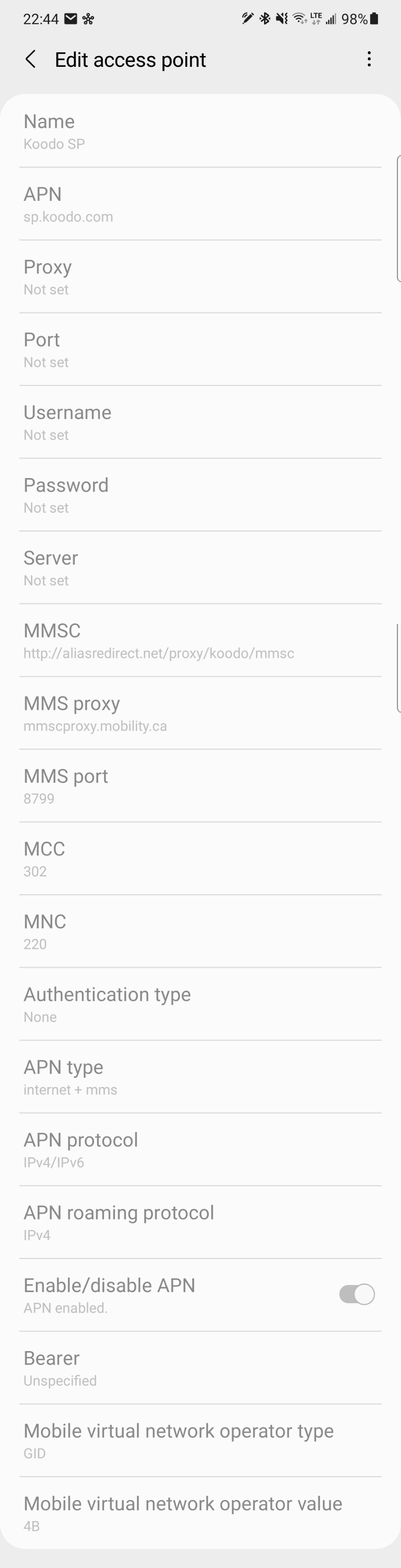The image is a cell phone screenshot of the "Edit Access Point" page. The title "Edit Access Point" is prominently displayed at the top center of the screen, slightly offset to the left, accompanied by a back arrow for navigation. Below the title, the page is divided into several editable sections detailing various network settings. They include:

- **Name:** KOODO.SP
- **APN:** SP.KOODO.COM
- **Proxy:** Not set
- **Port:** Not set
- **Username:** Not set
- **Password:** Not set
- **Server:** Not set
- **MMSC:** A web address is displayed underneath
- **MMS Proxy:** MMSproxy.mobility.ca
- **MMS Port:** 8799
- **MCC:** 302
- **MNC:** 220

Each setting is clearly listed, providing necessary information for editing the access point network configurations.